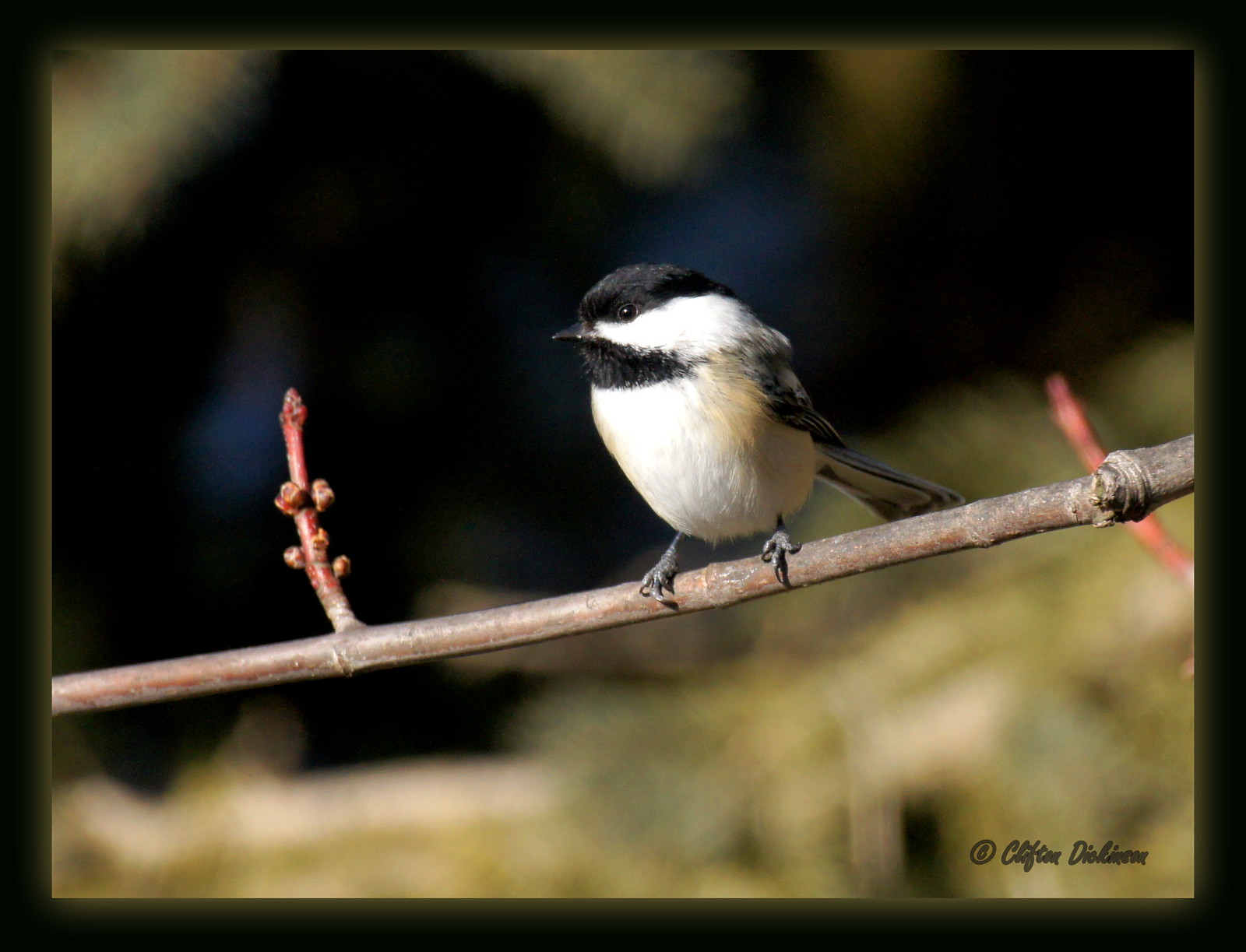This image features a small bird, specifically a black-capped chickadee, perched on a horizontally aligned branch that spans the width of the frame. The chickadee, positioned centrally and facing left, boasts distinctive markings: a white chest and cheeks, a black cap and throat, and black and beige wings. The branch, which is brown, hosts several red buds, suggesting that it's early spring and the tree is just beginning to bloom. A smaller twig with additional buds extends upwards from the main branch on the left side of the image. The background is artistically blurred, comprising shades of black, brown, and light green, which adds depth while keeping the focus on the bird and branch. In the bottom right corner, the text "Copyright Clifton Dickinson" is clearly visible, indicating the creator's ownership of the image.